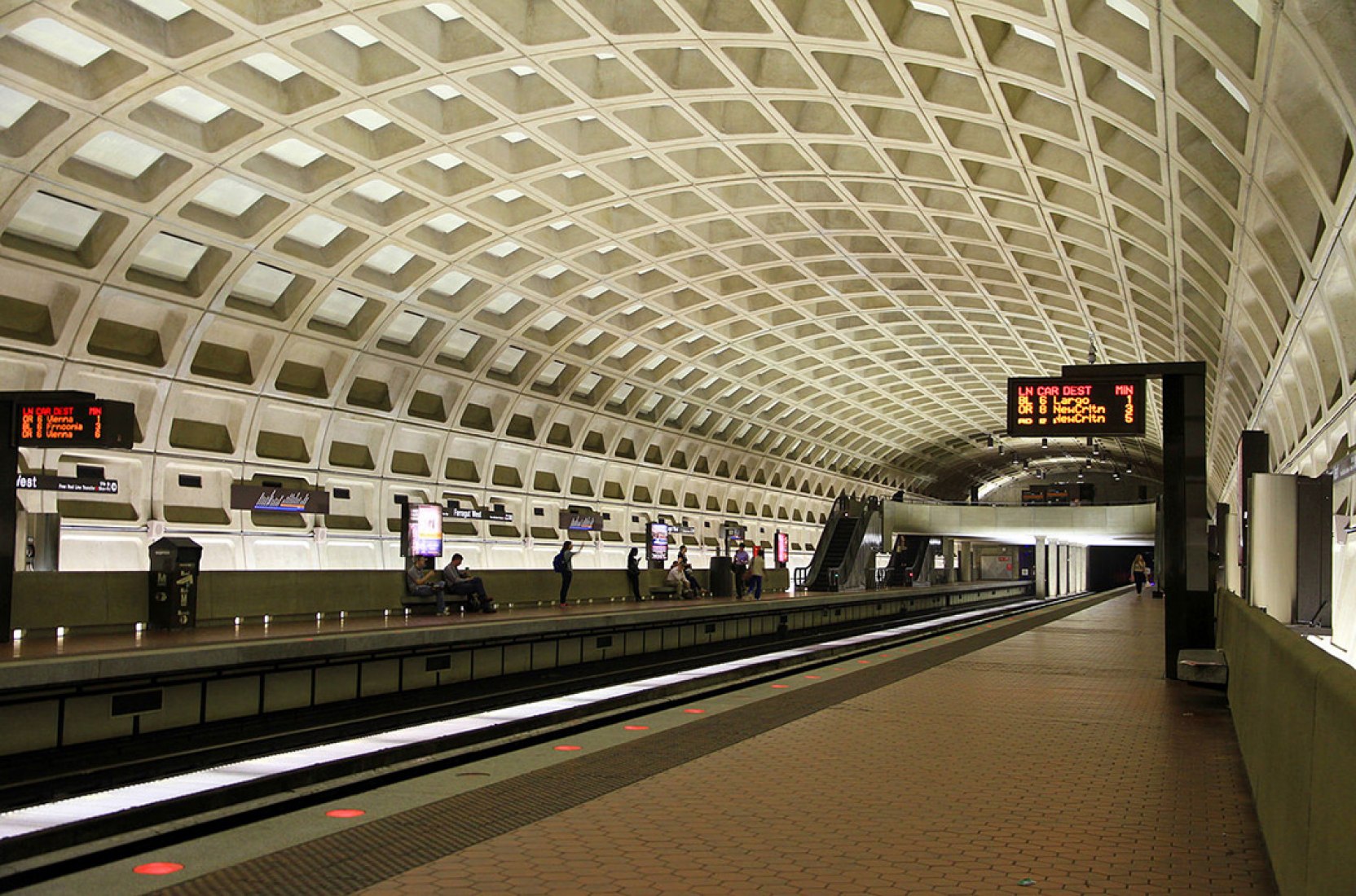The image captures a pristine subway train station, characterized by its clean and modern environment. The long hallway features a centrally placed track flanked by platforms where passengers are seated and engaged with their phones, waiting either to board or after disembarking from a train. The architecture is striking, with a dome-shaped, waffle-patterned ceiling that may be both structurally supportive and aesthetically pleasing. Electronic information boards display train schedules and updates. The platform edge is lined with sunken red lights, likely serving as safety indicators to warn passengers when a train is approaching. In the background, escalators provide additional access points. The overall atmosphere is orderly and well-maintained, devoid of any graffiti, trash, or disturbances.